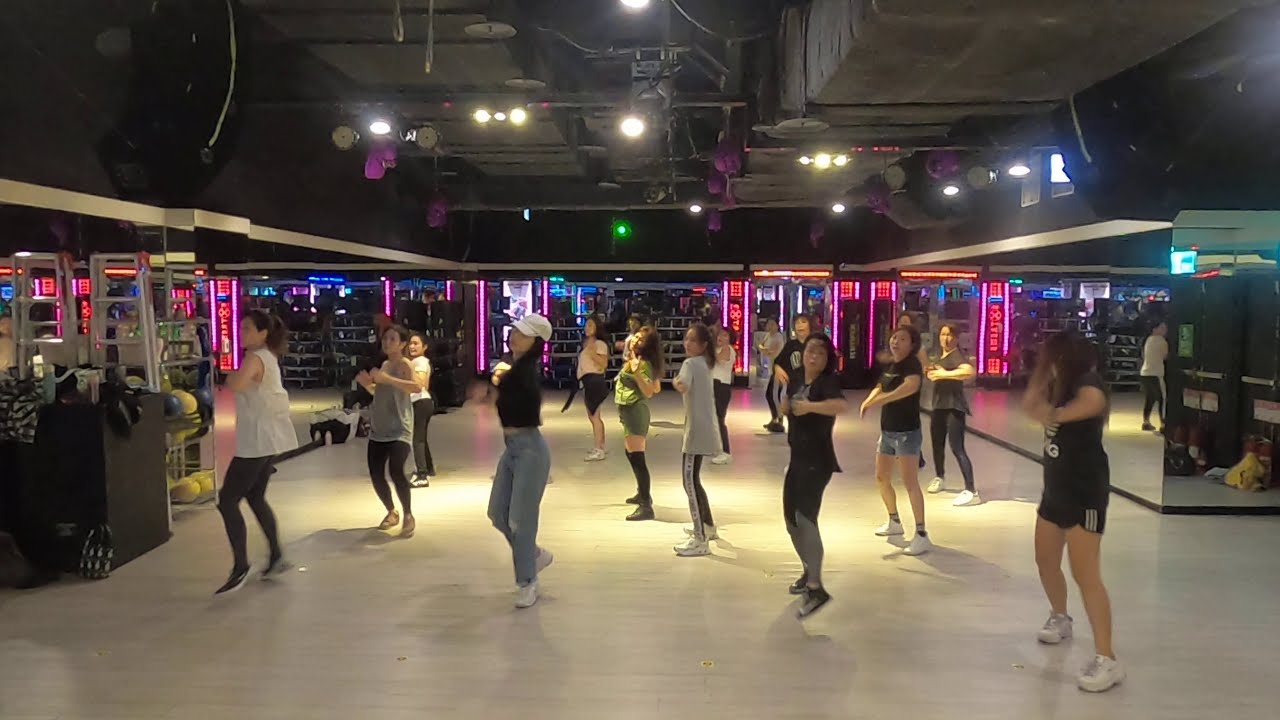The photograph captures the energetic atmosphere inside a bustling dance studio, featuring a white floor and a mirrored wall on the right side, which reflects the lively scene. The room is bathed in the glow of pink and red neon signs, and the back wall is adorned with shelves whose contents are unclear from this distance. Approximately 20 women, primarily Asian and ranging from young to old, are arranged in rows, intently practicing choreography. The majority wear athletic gear, but some sport more casual attire such as jeans and hats. Overhead, lights illuminate the high ceiling, enhancing the spacious feel of the studio. To the right, there is an assortment of open space, along with a bin of hats and bags and racks holding gym equipment. The left side of the image intriguingly hints at items that almost resemble bowling balls. The overall scene is vibrant, detailed, and brimming with the synchronized energy of the dancers.